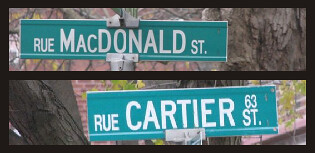This image is a detailed collage, presented in a rectangular landscape orientation, featuring two small photographs stacked vertically. Each photograph captures a standard mint-green street sign with white text. The top sign reads "Rue MacDonald Street," while the bottom sign reads "Rue Cartier Street 63." Both signs are mounted on traditional signposts, set against backgrounds that include a mix of greenery and possibly some houses, suggesting a suburban or urban environment. The use of the word "Rue" indicates that these signs may be from a French-speaking region, possibly Canada. The names "MacDonald" and "Cartier" are prominently displayed in large letters, denoting the street names in a clear and easily readable format.